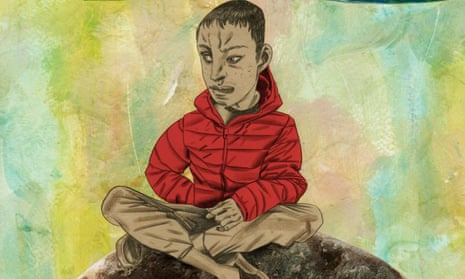The image is a detailed cartoon illustration of a man sitting cross-legged on a rock, facing the viewer but looking slightly to the left. His attire includes a red padded, long-sleeve hoodie with a front zipper and a hood, paired with tan pants that have a tight cuff around the shin. The man has a distinct appearance with short dark, unevenly cut hair, large eyes, tall and thin eyebrows, and a noticeable scowl on his face. His facial features are somewhat distorted and angular, reminiscent of a Picasso painting, giving him an almost Frankenstein-like, surreal quality. He wears brown slip-on shoes without socks. One of his hands is tucked into his coat pocket while the other hovers near his ankle. The background is a multicolored mix of white, blue, pink, and yellow shades, scarred and muted, adding a whimsical and textured backdrop to the scene.